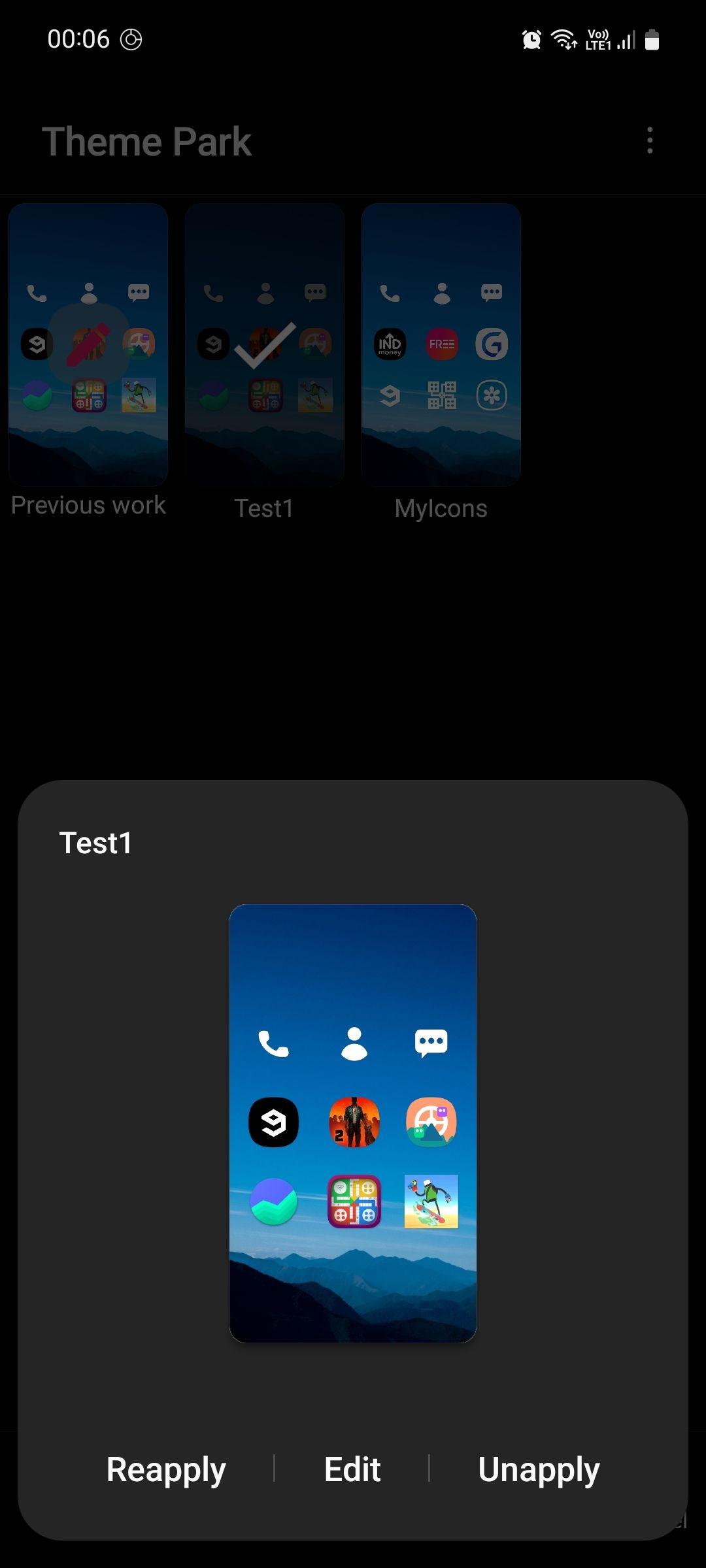The image is a screenshot from a mobile device. In the top left corner, there's a time display reading "00:06" alongside icons for an alarm and battery percentage. Below this, the background consists of a theme park image, though it is partially obscured by other elements in the foreground. At the top of the screen, white text reads "Theme Park."

Beneath this, there are three thumbnail images, each resembling a mobile phone screen. Below the left thumbnail, it is labeled "Previous Work," the middle one is labeled "Test Number One" and is checked, while the right one is labeled "My Icons." Each screen image is slightly different from the others.

At the bottom section of the image, the selection labeled "Test Number One" appears enlarged. The top portion reads "Test Number One" in white text. Below this, there is a close-up view of a mobile screen displaying nine icons: a phone icon, a person icon, a text message icon, and six game icons.

At the very bottom, there are three options displayed in white text: "Reapply" on the left, "Edit" in the middle, and "Unapply" on the right.